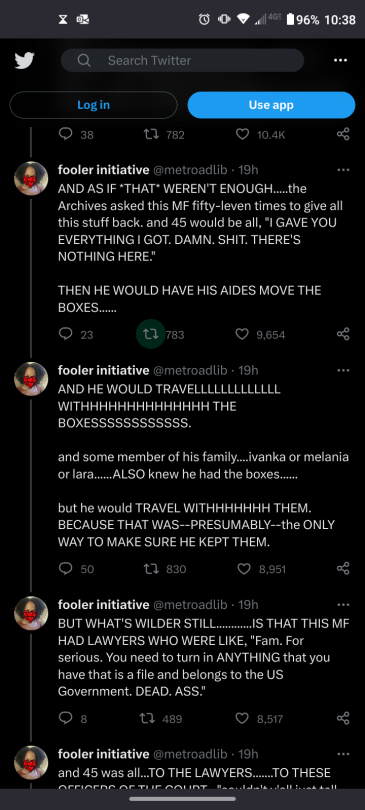This is a detailed screenshot of the Twitter app on a smartphone in dark mode, showcasing a sleek, black background. In the upper left-hand corner, the iconic Twitter bird logo is displayed next to a search bar with the placeholder text "Search Twitter." Below the search bar are two buttons: a login button and a prominent blue "Use App" button.

The main focus of the screenshot is a series of tweets from a user named Fooler Initiative. The user's profile picture features an individual with frizzy black hair and a red face mask. There are three tweets visible in their entirety, arranged from top to bottom:

1. "And as if that weren't enough, the archives asked this MF 5011 times to give all that stuff back, and 45 would be all, 'I gave you everything I got. Damn, there's nothing here.'"
2. "Then he would have his aides move the boxes, and then he would travel with the boxes."
3. "Some member of his family, Ivanka or Melania or Lara, also knew he had the boxes, but he would travel with them because that was presumably the only way to make sure he kept them."

These tweets delve into a narrative of persistent attempts by an authority to reclaim items, with a focus on the individual's evasive actions and involvement of family members.